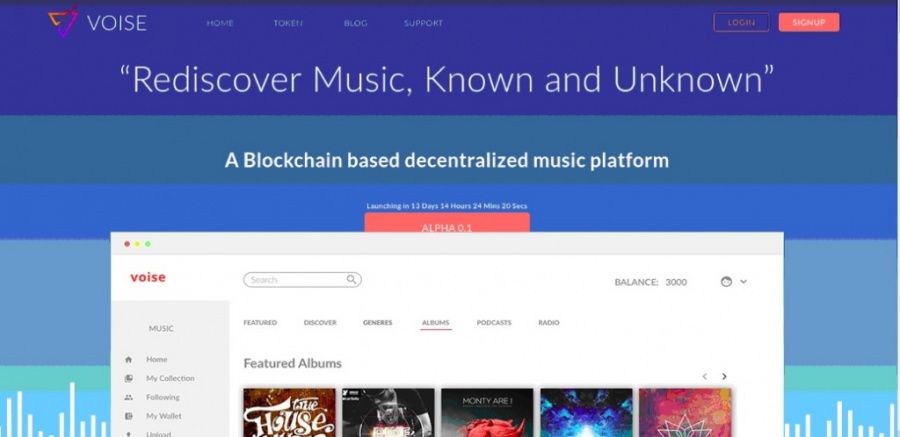The image showcases a screenshot of VOISE, a blockchain-based, decentralized music platform designed to help users rediscover music known and unknown. The platform seems to be presented in a clean, modern interface reminiscent of iTunes, with various shades of blue creating a visually appealing backdrop. Prominent features of the software interface include tabs such as Featured, Discover, Genres, Albums, Podcasts, and Radio, suggesting a wide array of content available for exploration. Additionally, options for personal customization are evident with sections like My Collection, Following, and Wish List located on the left side of the screen. The screenshot displays a selection of album covers, hinting at genres like metal and electronic, although their titles are not visible. Overall, the sophisticated design and wide array of functionalities imply a comprehensive platform for diverse musical interests.